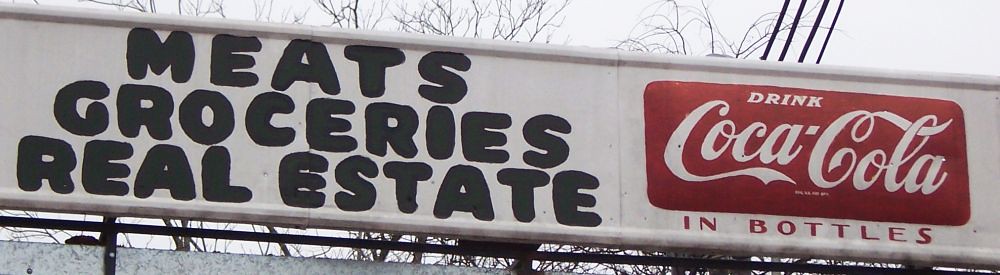In the image, a prominent white sign displays three distinct categories in bold black letters: "MEATS," "GROCERIES," and "REAL ESTATE." To the right of these listings, integrated within the same sign, is a vibrant red section that reads "DRINK COCA-COLA" in large, classic white letters, accompanied by the phrase "IN BOTTLES" beneath it in smaller red letters. The background reveals a couple of bare, leafless trees, adding a stark, almost desolate feel to the scene. Additionally, there are four visible cables or poles extending above the right side of the sign, contributing to the overall ambiance of the setting.